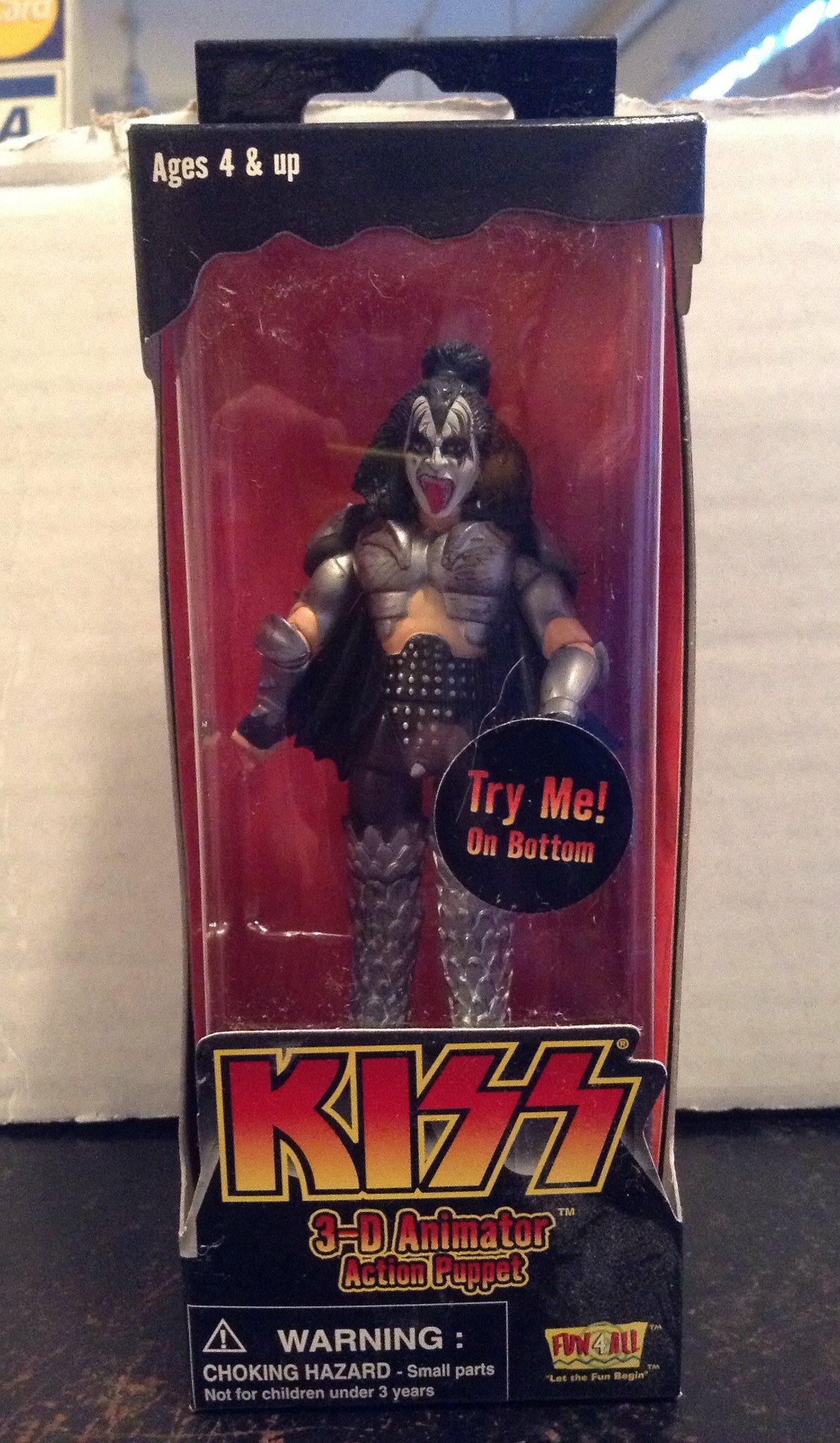This is a detailed close-up photograph of a collectible KISS figurine encased in a vibrant black box with a fiery red backdrop. The top of the packaging features large bold letters spelling "KISS" in a gradient of orange and red, outlined in yellow. Beneath that, in similarly styled lettering, it reads "3D Animator Action Puppet." The box prominently displays a "Try Me Button" sticker in a black circle with text starting in red and fading into yellow, complete with an exclamation mark. The figurine inside dons the iconic KISS makeup: a white painted face accentuated with black designs, including dramatic lines around the eyes, black eyeshadow, and a protruding red tongue. The character has long black hair, partially tied up in a bundle at the back. He is clad in a striking silver costume with metallic elements—silver arm covers, chest plate, and pants that transition into black near the cuffs. The packaging details include a cloud-like white border declaring "Ages 4 and up" and a cautionary rectangle with a yellow triangle exclaiming, "Warning... Choking Hazard - Small parts not for children under 3 years old." Additionally, there's a logo featuring a yellow trapezoid with red text that says "Fun 4 All" followed by "Let the fun begin™." The whole ensemble appears to be shot against a scratched, dark wooden countertop beside a white cardboard shipping box.